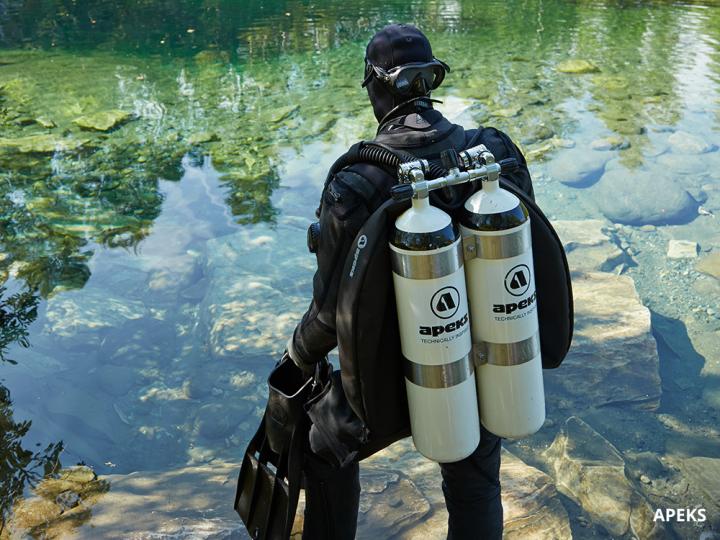In this detailed close-up photograph, a scuba diver is captured preparing to enter a body of clear, shallow water. The diver is fully equipped in a black diving suit with a mask and goggles, which are currently worn backwards with the eyepieces resting on the back of his head. He is equipped with two white air tanks mounted on his back, connected by two metal rings and a tube. Both tanks feature the word "APEX" in black text above a black logo, and the words "TECHNICALLY" and "TECHNOLOGY" written beneath it.

The diver is gripping his fins in his left hand while examining the water below. The rocky underwater terrain is clearly visible, suggesting a potential underwater cave or other rocky formation. The reflection of trees gives the water a greenish hue. Additionally, in the bottom right corner of the image, there's a white text watermark reading "APEX" (A-P-E-K-S).